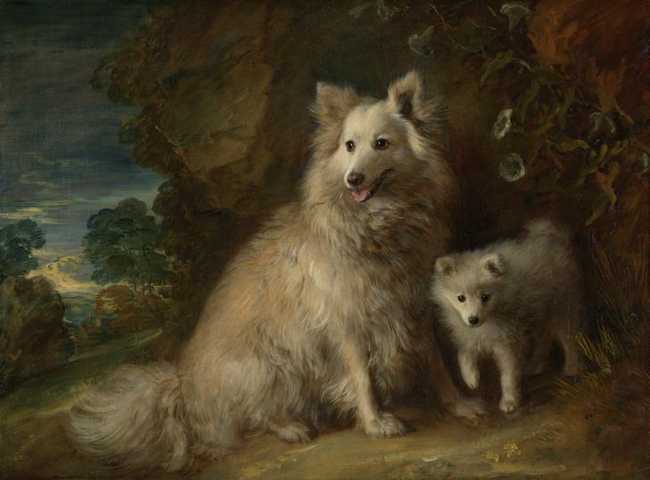This painting depicts a serene outdoor scene featuring a mother dog and her pup, both with thick, white fur. The mother, a large and very fluffy dog, is sitting on her haunches with her front legs bent in a protective stance. Her sharp nose, black eyes, and pink tongue sticking out add character to her expressive face, and her fluffy tail is visible to the lower left of the image. Standing close to her, near one of her legs, the smaller puppy mirrors her appearance with bent ears and a curled tail. The pup, more focused towards the viewer, has one paw raised in an inquisitive manner.

The background is rich with natural elements, dominated by earthy browns, muted blues, and touches of orange and green. Trees and bushes form a dense backdrop, with the sky peeking through the foliage towards the upper left. This earthy palette enhances the tranquil setting and complements the dogs' pristine white fur. The scene, subtly slanted, encapsulates a moment of protective affection amidst nature, drawing attention to the tender bond between the mother and her pup.